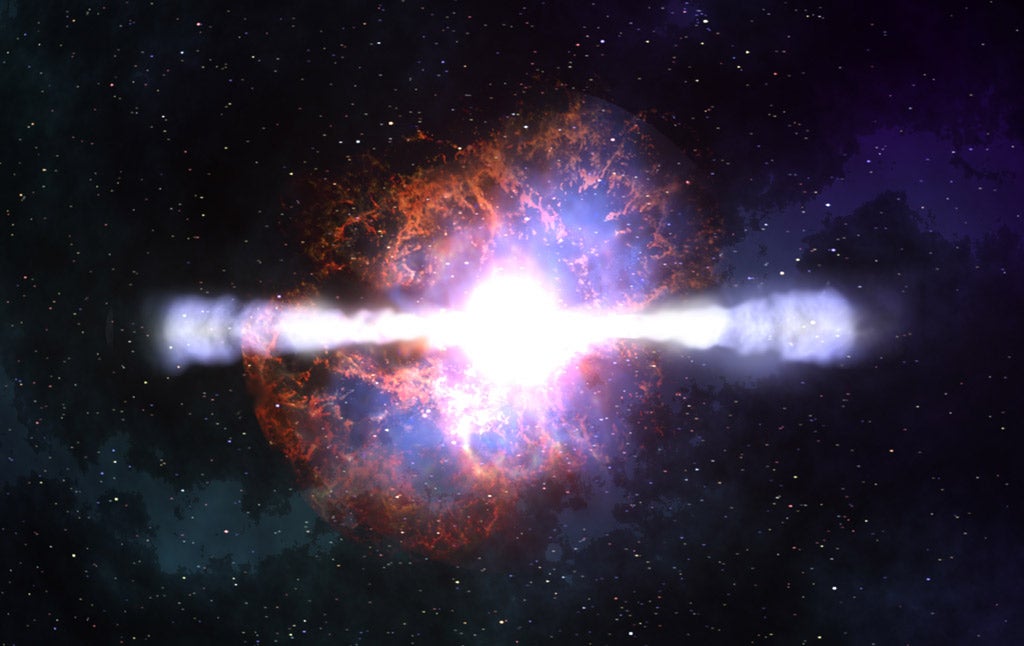This digital or artist's representation of a cosmic event in outer space showcases what seems to be a supernova or star explosion. At the heart of the image lies a brilliant, almost blinding white core, radiating intense light with reflections extending outward, forming glare on both the left and right sides. Enveloping this luminous center is a round formation of swirling orange and blue gaseous clouds, creating a spectacular, circular nebula. These gases appear to flow outward, gradually diminishing in brightness as they extend further from the core. The nebula's outer edges are surrounded by dense, dark space punctuated by twinkling stars, adding to the grandeur of the scene. Among the countless stars, there are variations in color, with some stars displaying hints of yellow, pale red, or pale blue. The background also features subtle fields of purple and turquoise, enhancing the richness and depth of the cosmic setting.